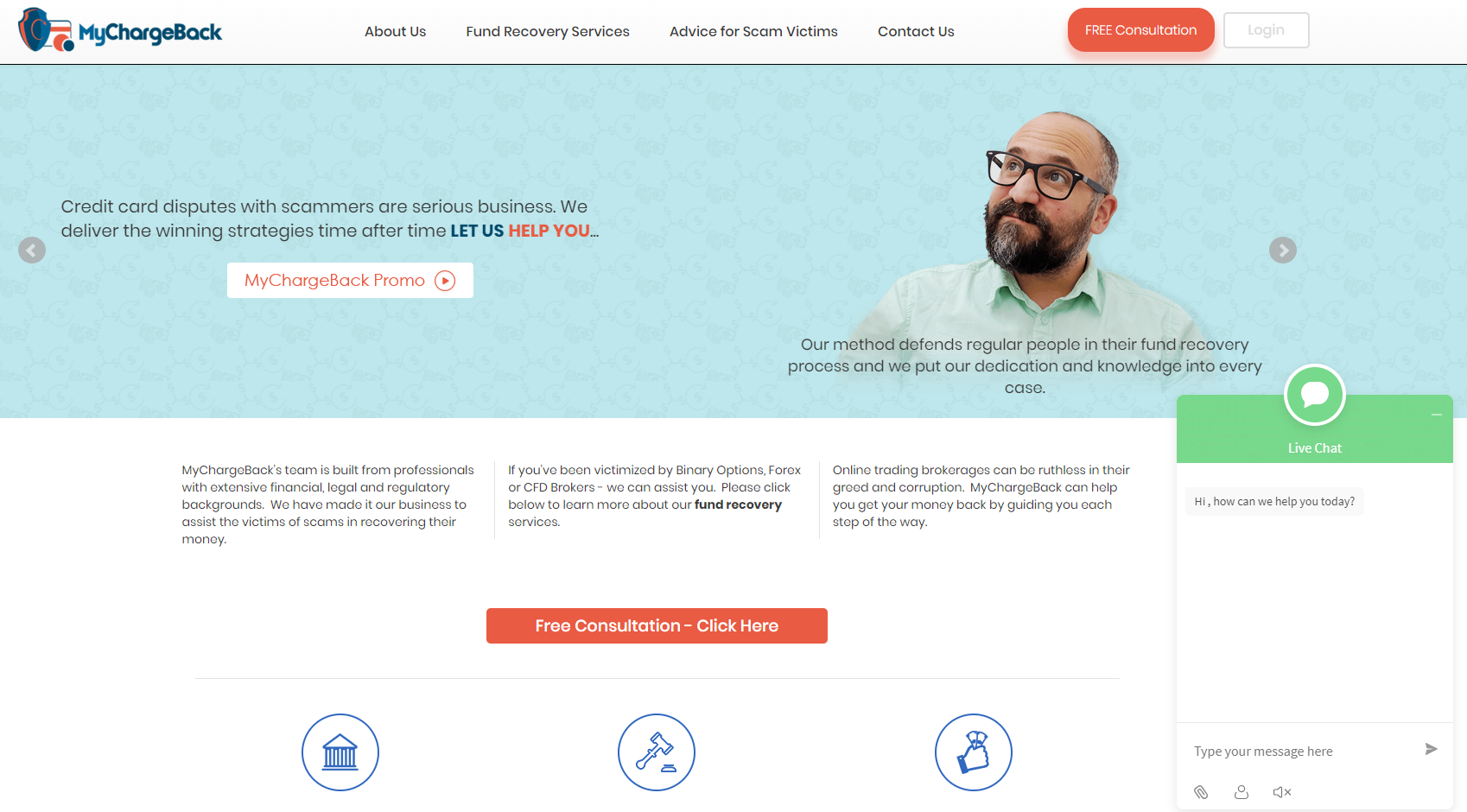Displayed on the screen is the MyChargeBack website, showcasing various sections including "About Us," "Fund Recovery Services," "Advice for Scam Victims," and "Contact Us," with options to "Login" or schedule a "Free Consultation." Prominently featured in the center is a light blue box. To the right of this box, there is an image of a gentleman with neatly cropped hair, dark black glasses, and a full beard and mustache, looking thoughtfully towards the upper right.

To the left of the gentleman, bold text reads, "Credit card disputes with scammers, a serious business. We deliver the winning strategies time after time," followed by "Let us help you," with an option to click on a "MyChargeBack Promo." Below the image of the gentleman, the caption states, "Our method defends regular people in their fund recovery process, and we put our dedication and knowledge into every case." Additionally, there is an active live chat feature on the right side of the screen, along with three brief informational points.